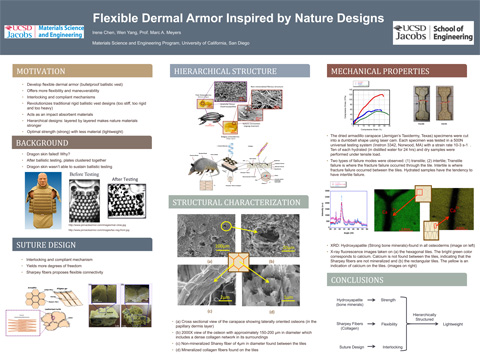The image is a detailed page, possibly from a textbook or a scientific chart, focused on "Flexible Dermal Armor Inspired by Nature Designs." At the top, there's a gray banner displaying the title in white text, flanked by logos for UCSD Jacobs Materials Science and Engineering and UCSD Jacobs School of Engineering. The page is divided into several sections, each with its own distinct, colored banner and corresponding content.

1. **Motivation**: On a tan background, this section appears to house a bulleted list, too small to read, but suggests reasons behind the study.
2. **Background**: Highlighted with a brown banner, this includes a bulleted list and three photographs.
3. **Suture Design**: With a grayish-blue background, this portion has a list, photographs, and what appears to be a hand-drawn image.
4. **Hierarchical Structure**: A gray banner introduces this section, which includes both labeled drawings and photos.
5. **Structural Characterization**: Set against a green background, this section shows four marked photographs (indicated with yellow arrows) alongside a detailed bulleted list.
6. **Mechanical Properties**: Identified with a brown banner, it features a chart depicting an upward trajectory in red, blue, and green lines, supplemented by images and another bulleted list.
7. **Conclusions**: On a light gray background, this final section includes a flow chart where smaller arrows converge into a single large arrow pointing right, summarizing the findings.

Each section aims to convey complex ideas through images and bulleted lists, although much of the detailed text and smaller elements remain too indistinct to read.